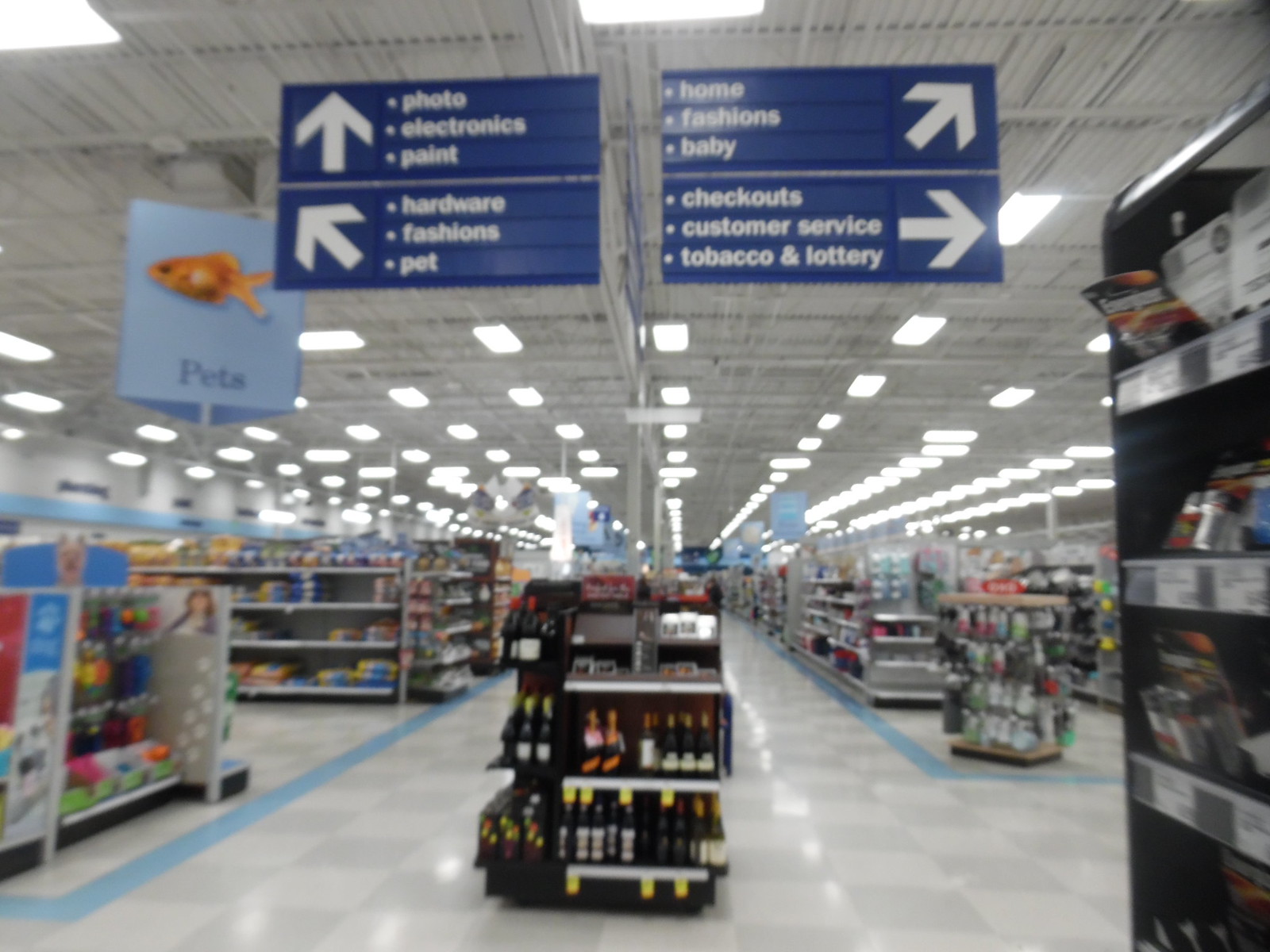In this image of a large department store, a wide-angle shot captures a bustling main aisle flanked by well-stocked shelves and a checkerboard-patterned floor in light gray and white. Along the floor, strips of light blue lines delineate the edges of the shelves. The bright white ceiling, illuminated by fluorescent lights, holds several directional signs. On the left, a notable teal blue sign depicting a yellow goldfish and labeled "Pets" marks the pet section. Above, there are directional signs in blue with white lettering: one with an arrow pointing up indicates "Photos, Electronics, Paint"; another with a left-pointing arrow reads "Hardware, Fashions, Pet"; to the right, two signs direct shoppers to "Home Fashions, Baby" and further right to "Checkouts, Customer Service, Tobacco, Lottery". Prominent displays include a battery rack showcasing Energizer products on the right and a central wine display featuring bottles on a darker-colored rack. Overall, the store appears spacious, well-lit, and organized, though a few shelves on the left side show some missing items.